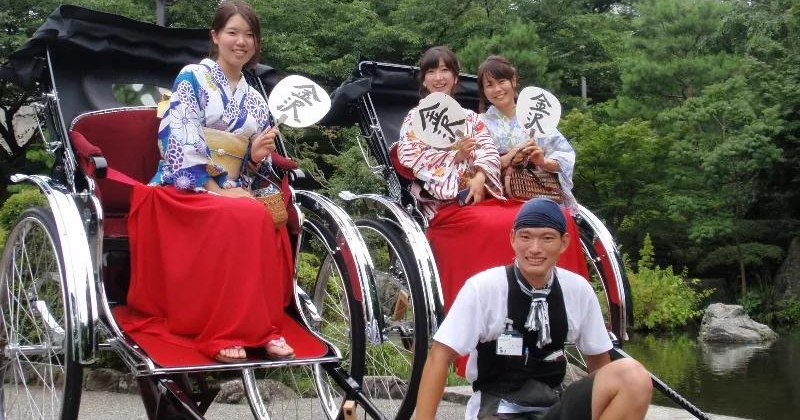The photograph captures an outdoor scene, likely set in Japan or China, featuring a picturesque backdrop of a serene lake surrounded by lush green trees and rocks. In the foreground, an Asian man, smiling and dressed in a white t-shirt, black vest, and black shorts, is crouching. He wears a blue bandana, a black and white scarf, and has an official name tag on his shirt.

Behind the man are two traditional rickshaws with distinctive high silver wheels, black canopies, and red seats covered by red blankets. The rickshaw on the left carries a woman dressed in a blue and white floral kimono, smiling at the camera while holding a white paper fan adorned with a large black Chinese character. The rickshaw on the right holds two women, each dressed in vibrant kimonos—one in red and orange, and the other in blue. Both women are also holding similar white paper fans with black characters and are smiling warmly at the camera. One of the women in the second rickshaw carries a brown purse. This image vividly captures a slice of cultural heritage amidst a tranquil natural setting.